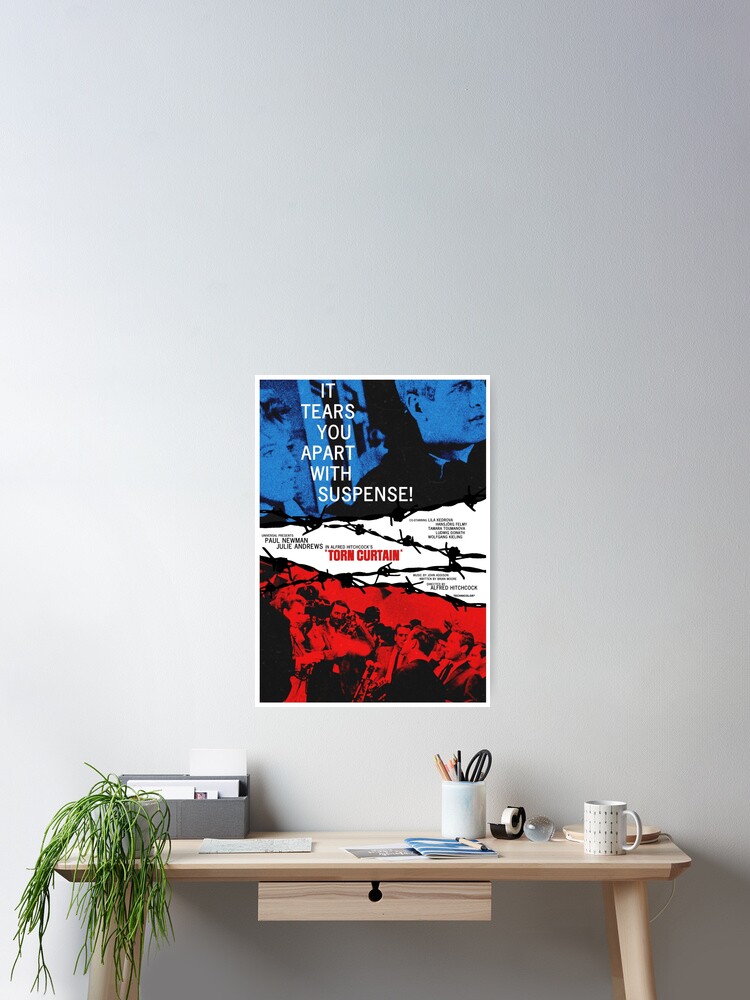This color photograph captures a small, meticulously arranged wooden desk positioned against a stark white wall. The desk, crafted from light-colored wood, features a single drawer with a distinctive keyhole-shaped black hole in its center, and stands on four circular legs that subtly splay outward at the bottom. Atop the desk, a white desk lamp with a bent neck casts focused light, highlighting a white cup mug filled with steaming coffee and a pencil holder brimming with scissors and pencils. A small roll of tape and some neatly arranged pamphlets also occupy the desktop space.

To the left side of the desk, a small potted plant adds a touch of greenery, with its stringy vines cascading over the desk's corner. A gray mail holder stands in the back left corner, organizing envelopes and papers.

Dominating the white wall above the desk is a vibrant movie poster, arranged in a tricolor theme with distinct sections: blue at the top, white in the middle, and red at the bottom. The top section features the gripping tagline, "It tears you apart with suspense." Below, the red title "Torn Curtain" stands out prominently in the white section. The poster features imagery of a man in a black suit and a woman's head highlighted in blue at the top, with red-toned figures dressed in black clothing below, enhancing the dramatic and suspenseful atmosphere it conveys.